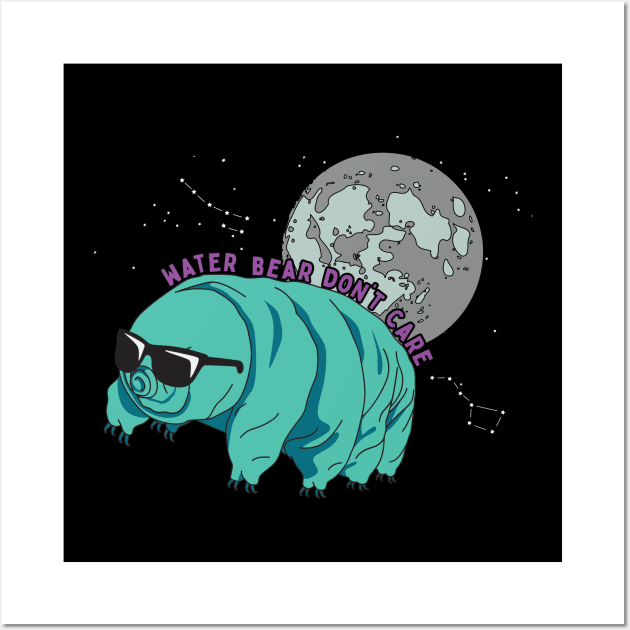This digitally created image is set against a white, square-framed background with a black interior, resembling a framed picture. The primary focus is a cartoonish, aqua-colored water bear (or tardigrade) with darker aqua claws and black sunglasses highlighted with a white glint. This whimsical tardigrade, which has four legs on each side and a pig-like nose, is floating in a space-themed setting. The text "water bear don't care" arches above the tardigrade in purple letters bordered in black, conforming to its shape. Behind the water bear, positioned slightly to the right, is a gray planet Earth with a bluish tint to the continents. The black background represents space, dotted with stars and the constellations of the Big Dipper to the right and the Little Dipper to the upper left.